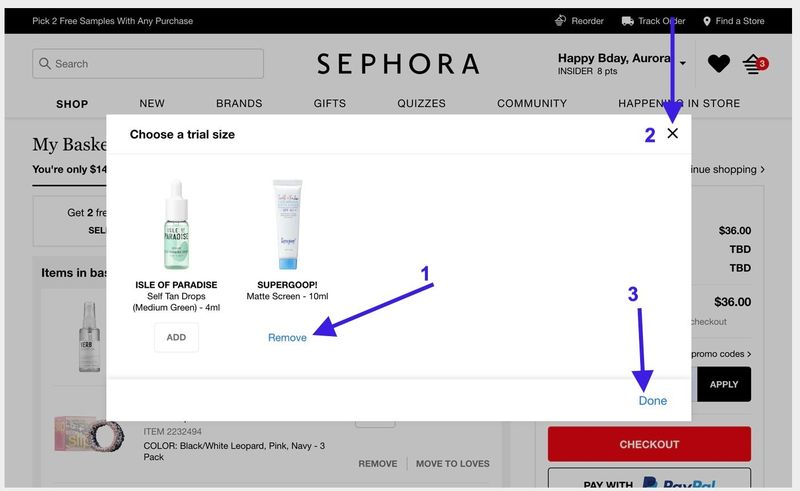This image is a screenshot from the Sephora website, indicated by the Sephora logo prominently displayed at the top center of the screen. The main focus is on a pop-up window in the middle of the image. The pop-up is a white rectangle featuring several elements. 

At the top left corner of the pop-up, the text "Choose a trial size" is displayed in black. On the top right, there's an X icon for closing the pop-up. A thin, horizontal line divides the window into sections. 

The midsection showcases two product options. On the left is "Isle of Paradise Self Tan Drops, Medium Green, 4ml" with a box labeled "Add" beneath it. To the right is "Supergoop! Matte Green, 10ml," with a box labeled "Remove" underneath it.

Three numbered, purple arrows highlight different interactive elements. The first arrow, labeled "1", points to the "Remove" option under Supergoop! The second arrow, labeled "2," points to the X icon at the top right of the pop-up, suggesting this as an exit option. The third arrow, labeled "3," points to the word "Done" at the bottom right of the pop-up.

In the background, at the bottom right corner of the image, the words "Checkout" and "Pay with PayPal" are visible, indicating additional steps in the purchasing process.